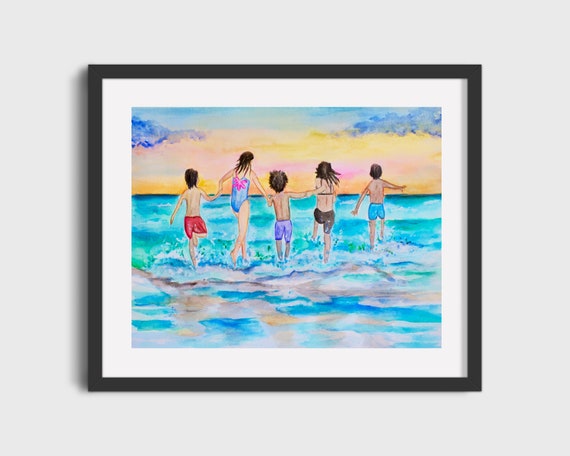The photograph captures a framed, hand-drawn piece of art mounted on a white wall. The artwork is encased in a black frame with an inner white border, emphasizing the vibrant scene within. The central image, likely rendered in watercolors, depicts five children joyfully playing in the ocean against a sunset sky, radiating hues of reds, pinks, yellows, and some blue clouds.

From left to right, the sequence of children includes:
1. A boy in red swim trunks.
2. A tall girl in a blue one-piece swimsuit, holding the first boy's hand and also the hand of the next boy.
3. A shorter boy in a purple swimsuit.
4. A girl, second tallest, in a brown two-piece swimsuit.
5. Another boy farther ahead on the right in blue swim trunks.

The children appear to be of Caucasian descent with varying degrees of tan skin. They are captured in mid-action, possibly running or splashing toward the crashing waves, embodying a carefree, joyous moment. The detailed and playful nature of the scene, along with the serene backdrop of a sunset sky and teal ocean waves, creates an atmosphere of warm, nostalgic summer fun.